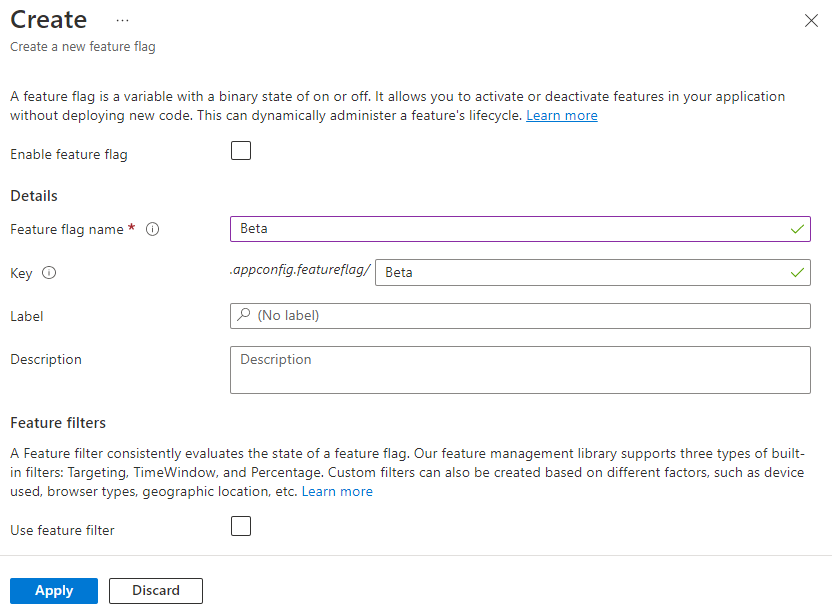The image depicts a screenshot of a website interface designed for managing feature flags within an application. 

At the top left corner, there is an option labeled "Create." Directly below this, a heading reads "Create a new feature flag," accompanied by a brief description: "A feature flag is a variable with a binary state of on and off. It allows you to activate or deactivate features in your application without deploying new code, enabling dynamic administration of a feature's lifecycle." There is also a "Learn more" link for additional information.

Further down, an option labeled "Enable feature flag" is presented with a checkbox next to it. Below this are detailed input fields for configuring the feature flag: 

1. **Feature Flag Name**: "beta."
2. **Key**: "beta."
3. **Label**: Currently, no label has been provided.
4. **Description**: No information is available here either.

Following these fields is a subsection titled "Feature Filters." It provides an explanatory note: "A feature filter consistently evaluates the state of a feature flag. Our feature management library supports three types of built-in filters - targeting, time window, and percentage. Custom filters can also be created based on different factors such as device used, browser types, geographic location, etc." There is another "Learn more" link in blue text for further reading.

Below this section, there is an option to "Use a feature filter" with another checkbox available for selection. 

At the very bottom left corner of the screen, two buttons are aligned side-by-side: 

- The first button is labeled "Apply" and features a blue background.
- The second button is labeled "Discard" with black text on a white background.